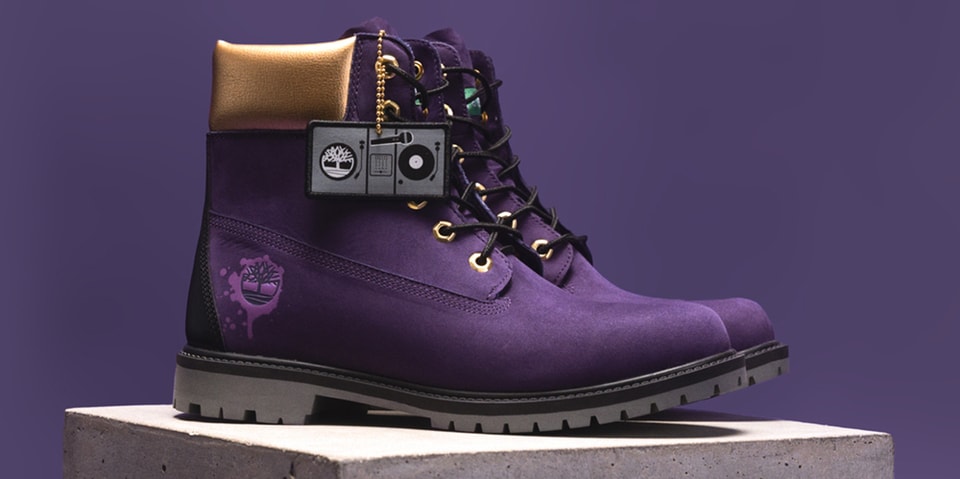The photograph presents a pair of dark purple Timberland boots prominently displayed atop a cement block. The background is a solid, dark purple-blue tone, enhancing the boots' rich color. The boots feature black rubber soles with non-slip grips, suitable for rugged use. They are detailed with metallic gold eyelets, resembling nuts and bolts, through which black laces are threaded. The padded cushioning around the ankles is also gold, providing comfort and a contrasting splash of luxury.

On the heel of each boot, a vibrant purple Timberland logo stands out. Dangling from each boot is a rectangular tag attached by a gold ball chain. This tag depicts a bird's-eye view of a DJ setup, featuring a vinyl record on a turntable, a record player arm, a square DJ mixer, and a microphone in the center. The detailed imagery on the tag complements the modern and stylish aesthetic of the boots.

These boots, shown in profile with their toes facing right, are showcased against the cement block and purple backdrop, emphasizing their trendy design and appealing to a fashion-conscious audience.